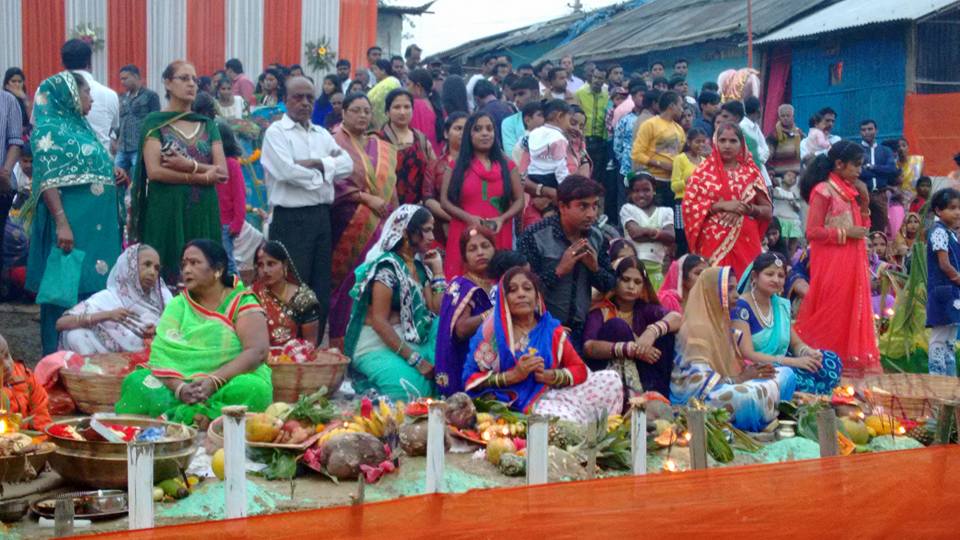The photograph captures a large gathering of Indian people, possibly celebrating an event such as a wedding or festival in a village setting. In the foreground, there are several weathered wooden poles, some painted white with peeling paint revealing the gray wood beneath. A small orange see-through fence is attached to these poles. Behind this fence lies a flat surface adorned with an array of bowls, plates, and fabric, all laden with various fruits and foods. 

Seated on the ground around these foods are mainly women, wearing vibrant traditional Indian saris and shawls in a spectrum of bright colors, including neon green, royal blue, magenta, and red. Many of them have their heads or shoulders draped with these shawls. The central woman, clad in a blue sari, has her hands clasped, appearing to be in prayer. In contrast, men are fewer but present, with some standing behind the seated women. One notable man dressed in a white shirt and pants stands out among them.

Behind the seated women, a mixed group of men and women stand in multiple rows, some holding small children. The scene is set against a backdrop of village buildings, including shacks with blue exteriors and one building with worn orange and white stripes and a red roof. The overall atmosphere is vibrant and communal, reflecting the essence of a traditional celebration.